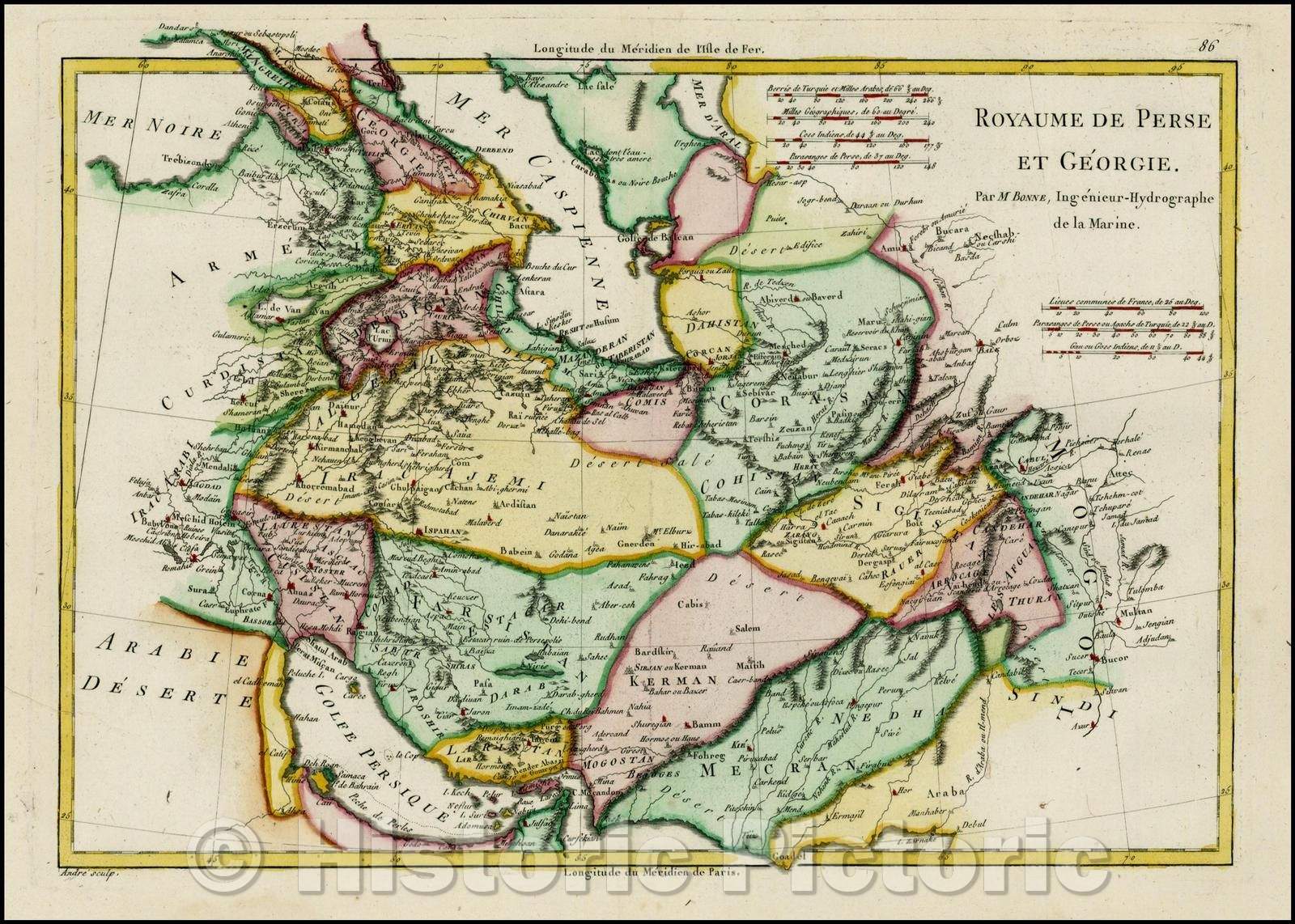This image depicts a detailed, vintage map with muted colors, predominantly featuring light green, light pink, yellow, and tan hues. The map, outlined by a yellowish gold border and framed by a light gray background with a black outline, appears to represent a region possibly within the Middle East. In the upper right-hand corner, the title "ROYAUME DE PERSE ET GEORGIE" is prominently displayed in black text, indicative of an older European language, likely French. Various country names such as Mercran, Kerman, and Perseque are labeled across the map, along with important geographical features like "Mer Noir" in the upper left and "Araby Desert" in the lower left. Scattered small black texts detail the regions further. At the bottom of the map, a translucent watermark reads "Historic Pictoric," emphasizing its antique nature. The map's subdued and timeworn appearance, along with diverse country regions shaded in yellow, red, and green, underscore its historical significance.